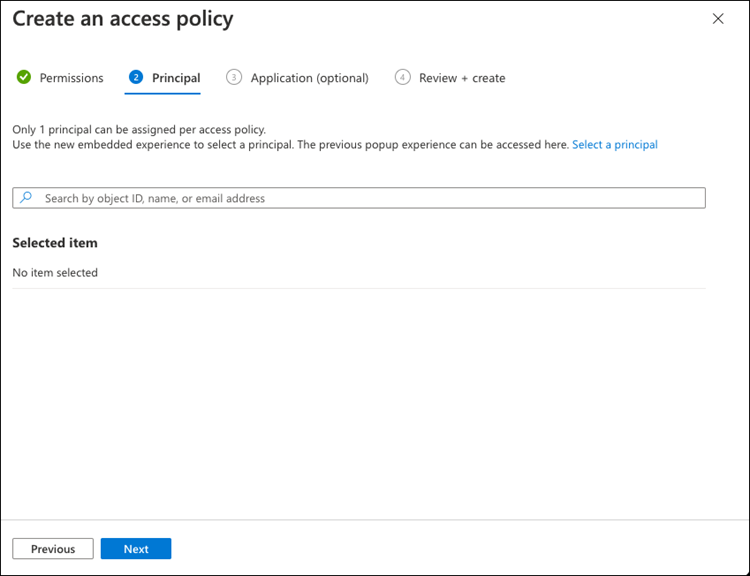The image displays a user interface of a website for creating an access policy. At the top left corner, there's an "X" icon for closing the window, while the top right corner shows the heading "Create an Access Policy: Permissions." 

The interface is divided into four steps, clearly indicated but focuses on the section where users assign a principal. Only one principal can be assigned per access policy. The instructions highlight an option to use a "New Embed Experience" to select a principal, along with a link in blue lettering that provides access to a previous pop-up experience. Users can search for a principal by "Object ID, name, or email address" using the search bar, which features a blue search icon.

In the "Selected Item" section, it is noted that "No item selected," followed by a large expanse of white space which dominates the screen. At the bottom of the interface, two buttons are visible; the "Previous" button is white and the "Next" button is blue.

Overall, the layout is clean and functional but lacks any visual flair or contextual information about the purpose of creating an access policy. It appears to be a step in a larger process but is otherwise plain and generic.